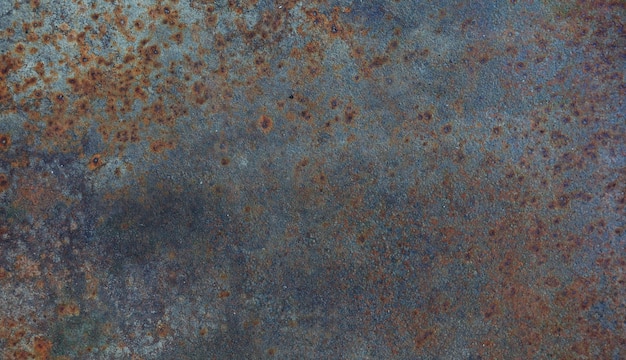The image appears to depict an abstract art piece or possibly a close-up of a rusted metal surface. The background is primarily a dark gray-blue or steel blue color, interspersed with light gray and white areas. Prominent splotches of what looks like rust in varying shades of brown, orange, and red are distributed across the piece, giving it an aged, weathered appearance. The left-hand side and top left corner display larger, more intense patches of rust, which fade out into smaller, more scattered spots as they approach the center. The central area and bottom middle remain mostly clear, revealing more of the blue-gray background. The right side of the image, particularly the upper corner and the length extending downward, features dense clusters of rust-like spots. Although the surface is reminiscent of rusted metal, the artful application and distribution of colors suggest it could be a painted representation, adding a layer of intrigue and ambiguity to the artwork.